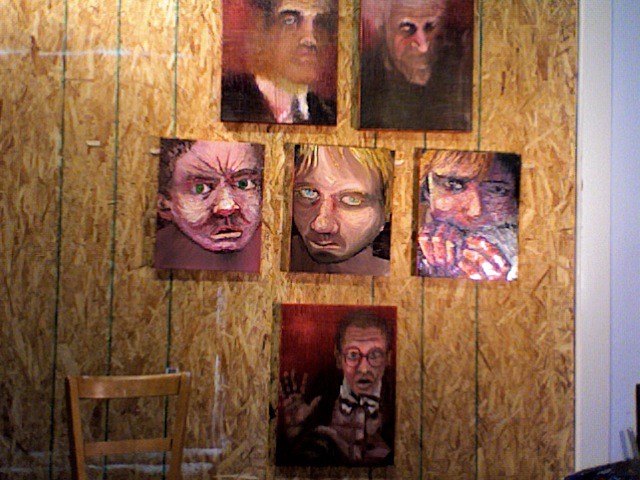The photograph captures an indoor setting featuring a rough, unfinished wooden wall with visible textures. Mounted on this wall are six slightly abstract, possibly amateurish, yet intentionally eerie painted portraits. Each portrait depicts a different person, primarily men, who all convey unsettling emotions. In the top left is a man with a blurry face, followed by an older man with no mouth in the next frame. Another ambiguous figure with lined features that could be either a baby or an adult adds to the disturbing aura. Additionally, there is a portrayal of someone, indeterminate as a child or adult, with hands to their mouth, and lastly, a man appearing horrified and shocked. Every portrait directs its gaze towards the viewer, amplifying the eerie atmosphere. Completing the scene, just beneath the portraits, the top of a light brown wooden chair is visible against the wooden backdrop, encapsulating the unsettling and enigmatic ambiance of the image.